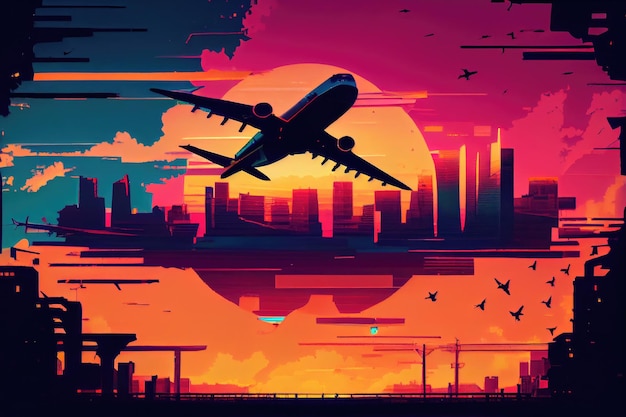The image is a detailed, rectangular artistic drawing, approximately four to five inches wide and three inches high, depicting an airplane in flight over a city. The composition is seemingly split into two distinct sections.

In the top half of the image, a black and blue airplane with a black underbelly and a blue top is seen rising diagonally from the lower left to the upper right, as if it has just taken off. The plane is set against a backdrop of a radiant yellow sun and shades of a pink, blue, and purple sky. The left side of the sky is primarily blue, transitioning to pink and purple with black birds flying on the right side.

Centered in the composition, stretching from the left to the right of the image, is a navy, purple, and pink city skyline with numerous skyscrapers. This skyline delineates the transition between the image's upper and lower halves and appears to be part of both.

In the bottom half of the image, a darker scene unfolds, characterized by a black walkway extending from the lower left to the lower right, bordered by structures resembling factory buildings. Above these structures rises an orange sky with birds, echoing the upper section's colors but in a more subdued, darker tone. Yellow smoke billows from the factories, scattering into the orange sky. Big power lines and other structures punctuate the scene. The sun's lower half appears again in this section but in purple, blending with the dark skyline above.

This detailed, vibrant drawing captures the contrasting elements of a bright sunset and a bustling urban landscape, split into dual perspectives that intricately connect the top and bottom sections.